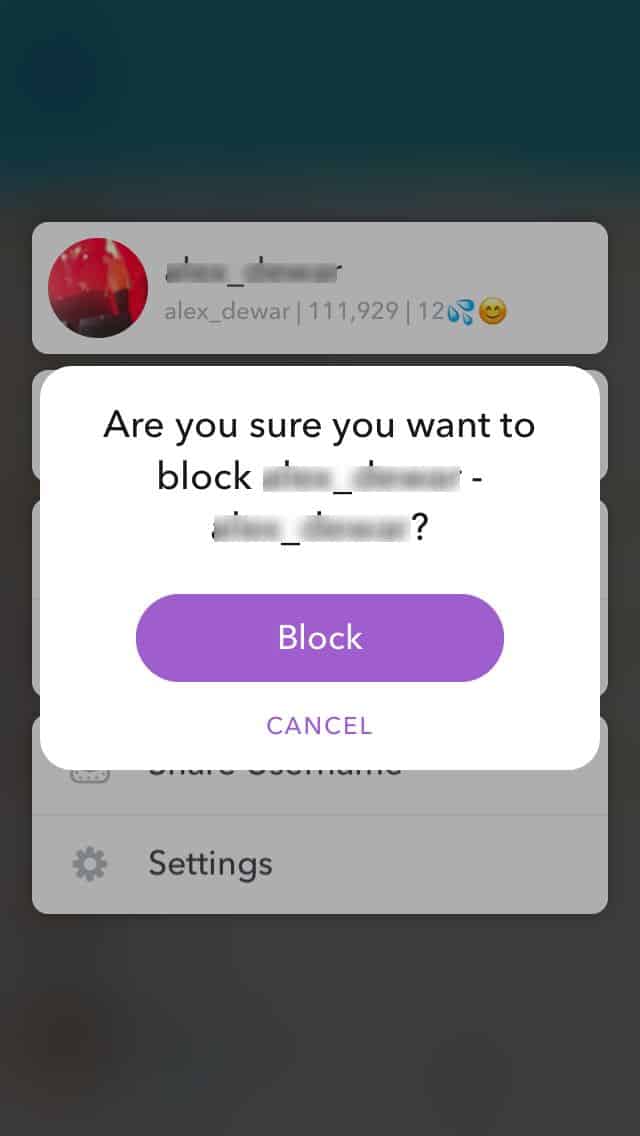Certainly! Here's a cleaned-up and detailed caption for the given image description:

"The image features a predominantly black background with the word 'block' prominently written in black text. Surrounding the word 'block' is a purple highlight, making it stand out against the otherwise dark backdrop. Additionally, there are small water drop icons and a smiley face emoji placed around the text. The background of the image also has distinct white areas, adding a contrasting element to the overall dark theme."